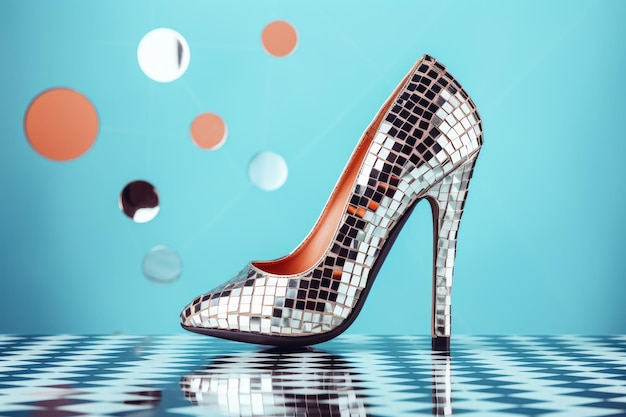A full-colored, square photograph captures a distinctly artistic composition with a striking focal point: a tall high-heeled shoe crafted from numerous tiny mirrors, resembling a disco ball. This shimmering shoe is positioned centrally on a checkered blue and white table. The backdrop features a blue wall adorned with variously sized circles, adding to the unique aesthetic. Among these circles are several in solid burnt orange, along with others in blue, white, black-and-white, and mostly black with a bit of white. The interplay of the reflective shoe and the visually dynamic background creates an intriguing, surreal scene.